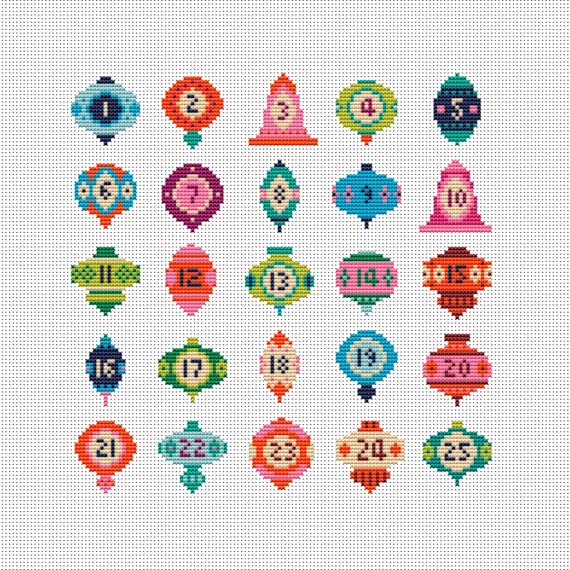This detailed work of art captures a counted cross-stitch piece on a white fabric background, showcasing 25 vibrant Christmas tree ornaments, each uniquely numbered from 1 to 25 in black. Arranged in five horizontal rows of five, these ornaments display a delightful variety of shapes, including bells, an object resembling an upside-down genie lamp, and others that echo the forms of skyscrapers or traditional Christmas balls. The colors range broadly, featuring shades of blue, orange, pink, green, yellow, and red. Each shape is meticulously detailed, such as the pink ornament with green tops and bottoms, the navy blue one with light blue spots, and an orange ornament with white accents. The numbered ornaments are crafted with different patterns and tones, creating a kaleidoscope of festive imagery that highlights the intricate artistry involved in this cross-stitch masterpiece.